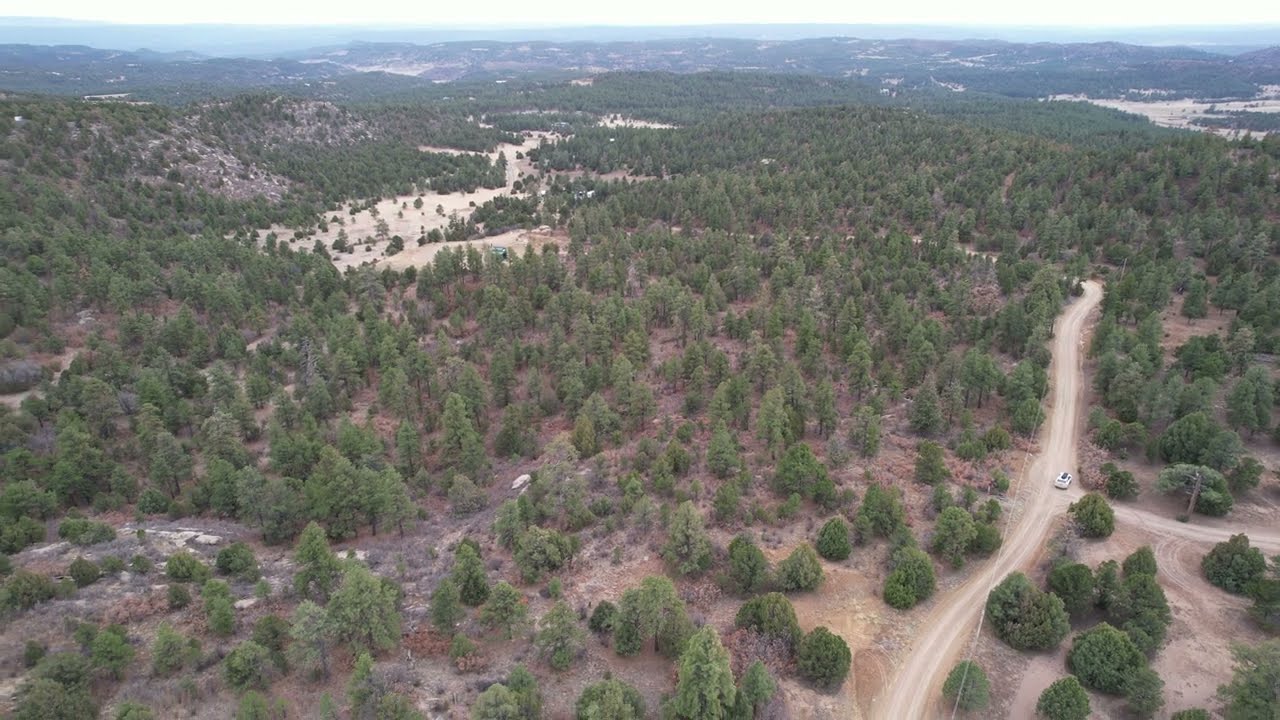This high-definition, landscape-oriented color photograph, captured from above by a drone, depicts a rural area characterized by its earthy tones and natural features. The scene is dominated by brown dirt roads cutting through a landscape dotted with short, scruffy pine trees. A key feature of the image is a dirt road that extends from the bottom right, leading to a T-intersection near the center where a vehicle is visible. This primary road takes a sharp left before disappearing into a wooded area and re-emerging in the top left section of the photograph. In the distant top right, a body of water such as a river or creek adds a touch of blue to the predominantly brown and green palette. Beyond the immediate roadways and trees, the terrain shows subtle variations in height, with low-lying areas and gentle slopes contributing to the overall rural and almost semi-desert appearance. The clear blue sky and distant mountain peaks create a serene backdrop, completing this detailed and realistic representation of a tranquil, country landscape.